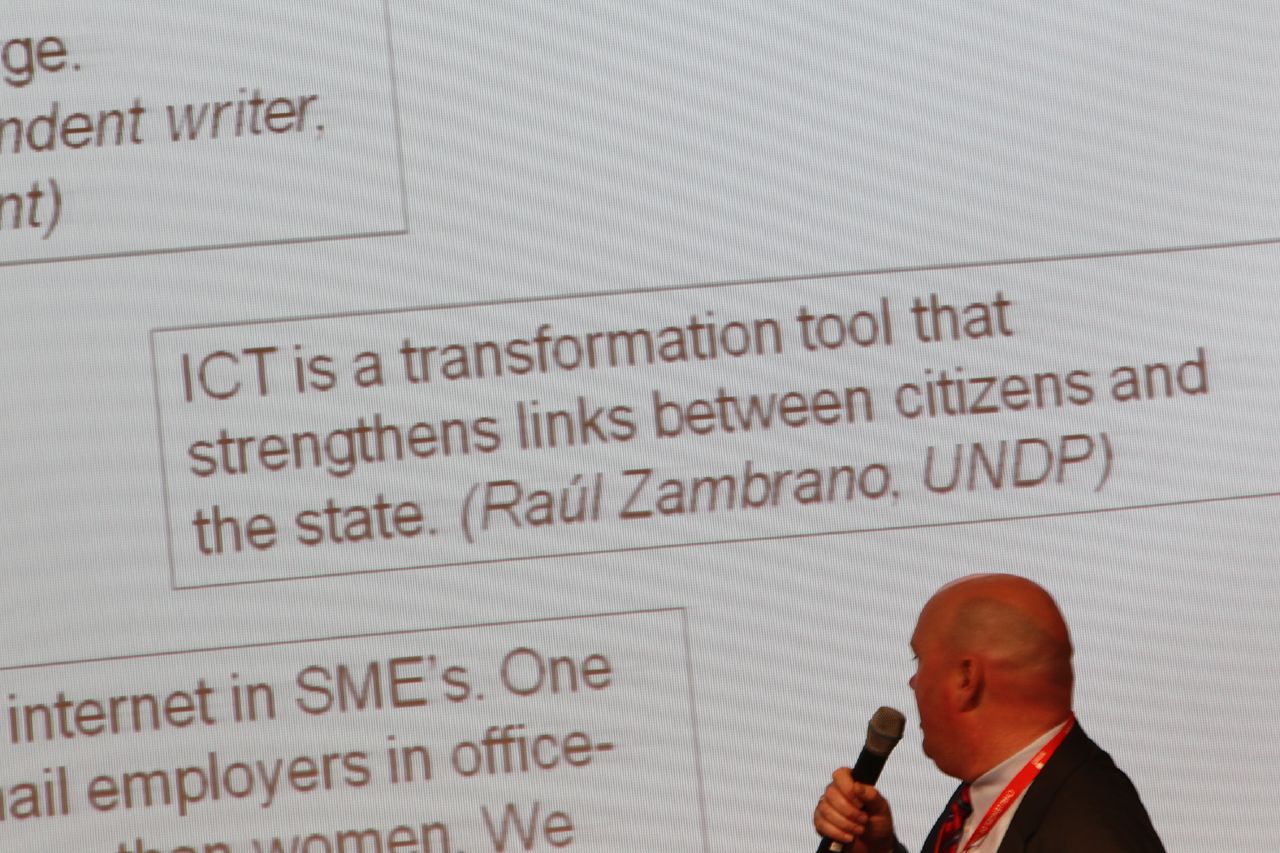The photograph depicts a balding man in a black suit and red tie, facing sideways but looking behind him at a projection screen. He holds a black microphone with a silver top in his right hand, which is the only part of his arm visible. He wears a white dress shirt and a red lanyard around his neck. The screen behind him has a white background with black text in various boxes. In the top left corner, there is black text that reads "G.E. ND NT Writer, NT," though it's partially cut off. Another box extends from near the center of the screen almost all the way to the left, containing the text: "ICT is a transformation tool that strengthens links between citizens and the state. (Raul Zambrano, UNDP)." Additional text boxes in the bottom left corner are partially visible, displaying fragmented words including "Internet," "employers," and "office." The layout suggests the man is likely presenting or addressing an audience, emphasizing the role of ICT in connecting citizens with the state.